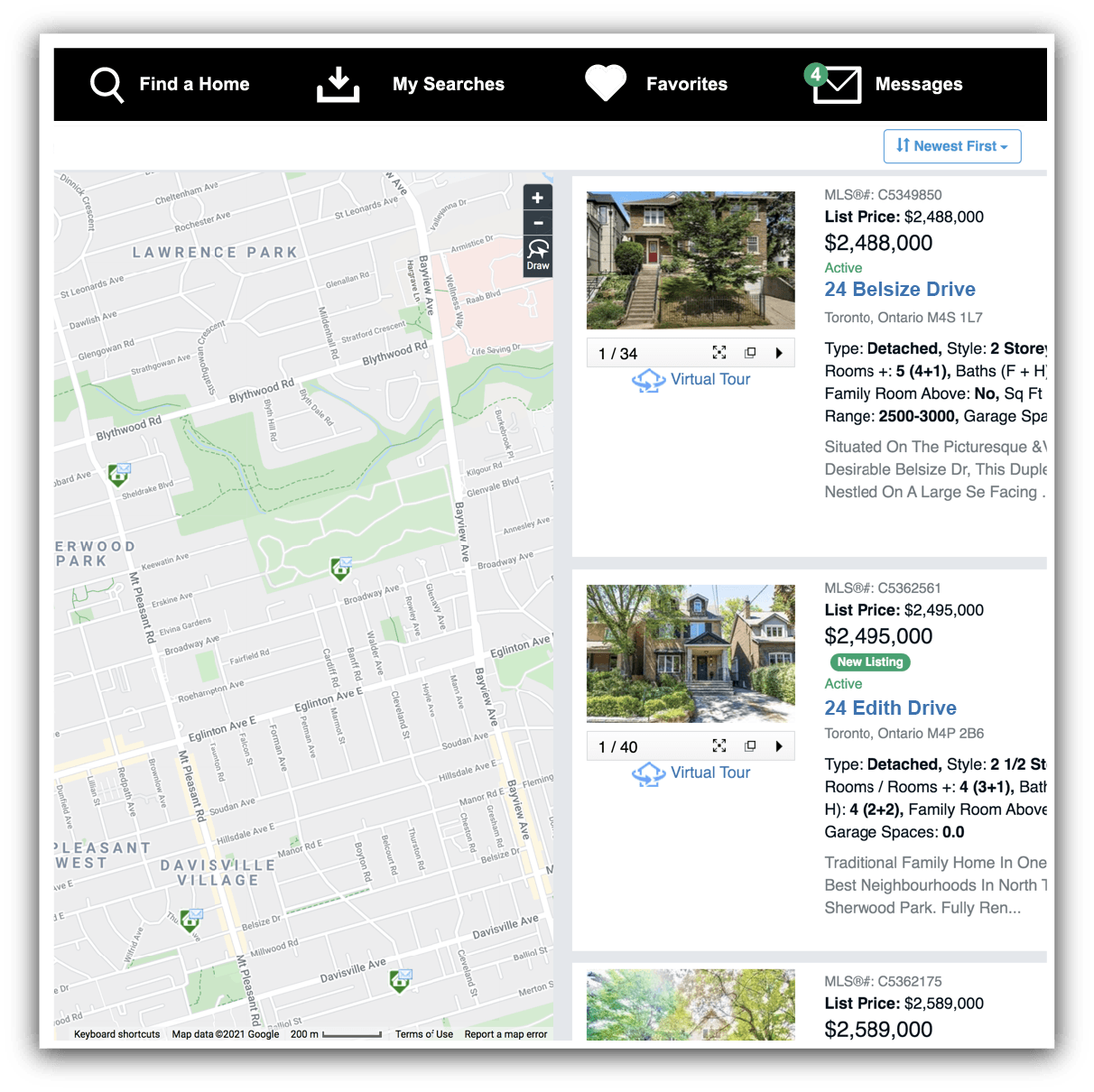The top section of the screen features a black navigation bar with options labeled "Find a Home," "My Searches," "Favorites," and "Messages." An envelope icon next to the "Messages" option indicates that there are four unread messages. On the left side of the screen, a Google Maps-like interface displays an area in Toronto, highlighting neighborhoods such as Lawrence Park and Davis Village.

On the right side, there are visible listings for homes. The first listing shows an image of a house with a front yard tree. The house is elevated, requiring several steps to reach the front door, while the garage is located at the ground level. This property is listed at $2,488,000 and is situated at 24 Belsize Drive, Toronto.

The second visible listing below features another house priced at $2,495,000, also located in Toronto, at 24 Edith Drive. These two listings are part of a broader search likely focused on the Toronto area. A third listing is partially visible, suggesting additional properties are available for viewing.